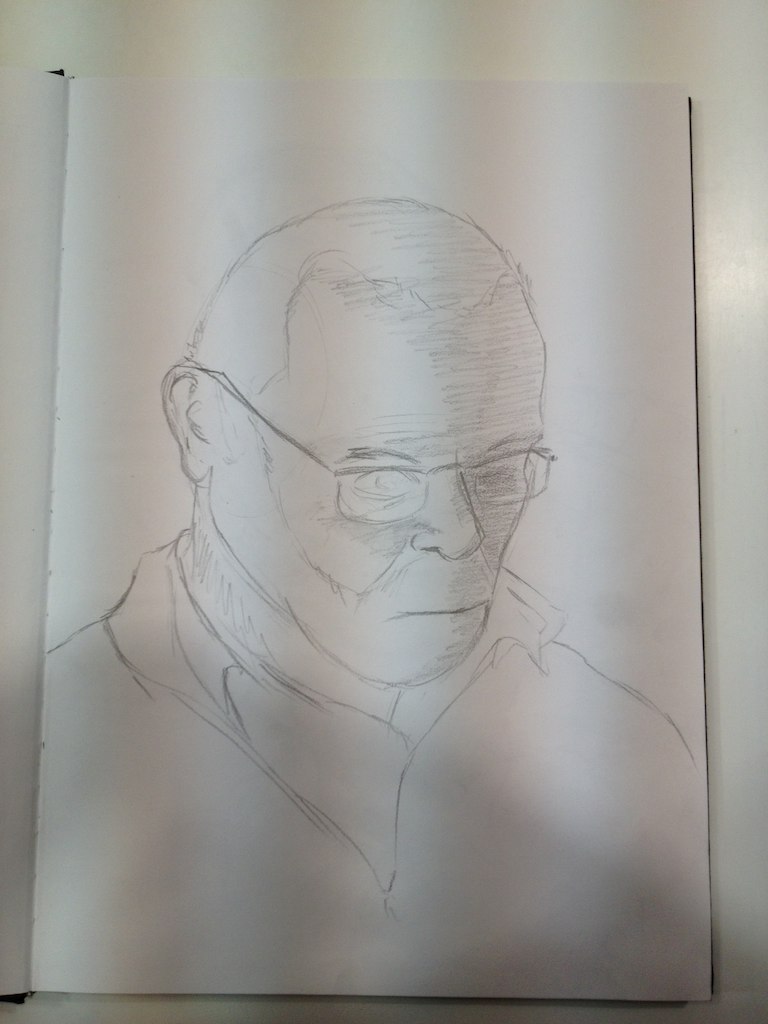The image depicts a detailed pencil drawing on a piece of white paper set against a white wooden background. The subject is an elderly man with a widow's peak hairline, closely cropped around the ears, giving the impression of a receding hairline. He wears wire-framed, rimless glasses that resemble almost "granny-style" glasses, adding a subtle charm to his appearance. His mouth is a thin, straight line, giving him a somewhat grim demeanor. The man is dressed in a turtleneck with a collared shirt over it, possibly made of velour, suggesting warmth and comfort. The bust-length portrait captures the man looking towards the bottom right of the image with meticulous pencil strokes, making it appear as though he might have drawn it himself.